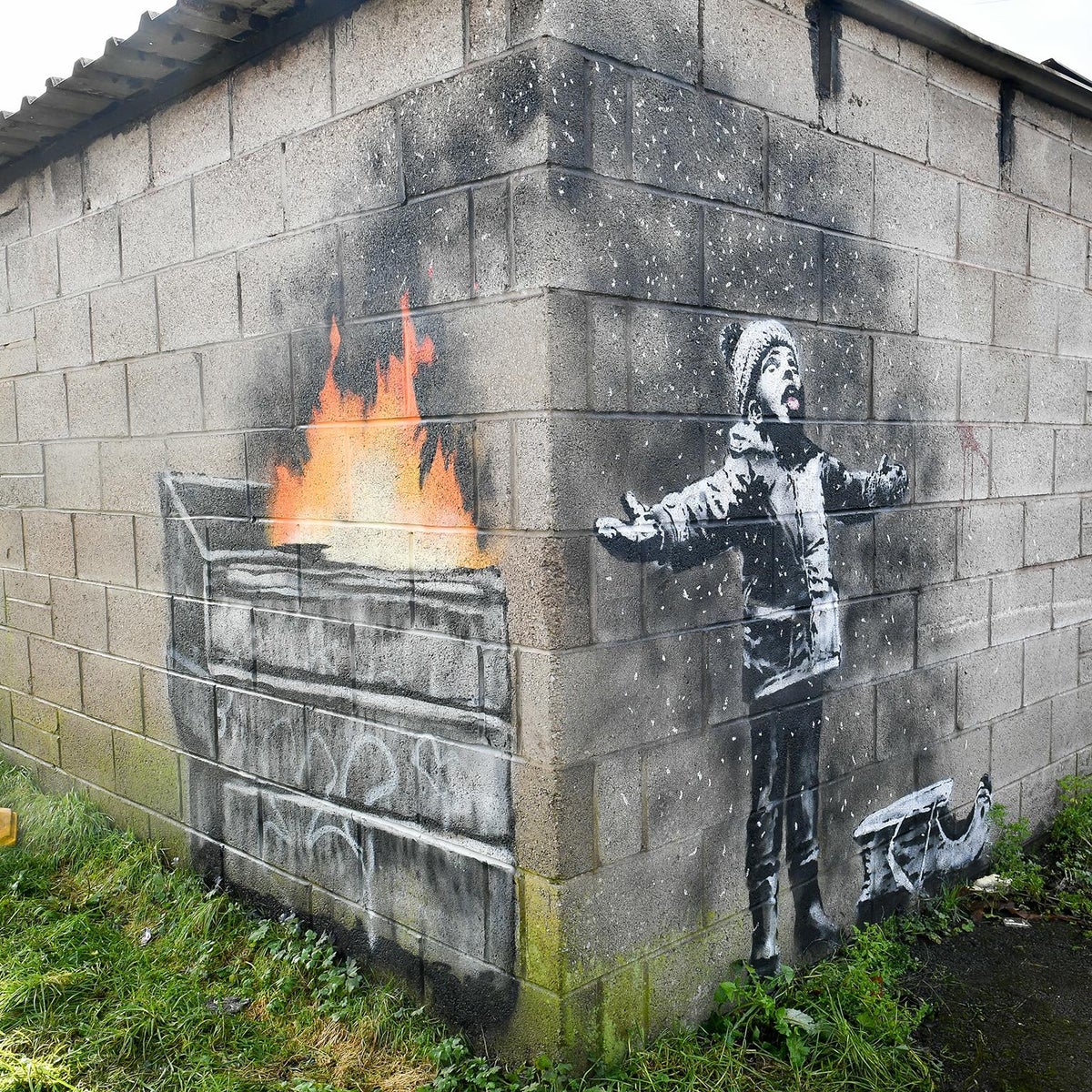In the corner of a stone building with cement blocks, there is a striking piece of street art that evokes the renowned style of Banksy. On the left side of the corner, there's an illustration of a gray dumpster engulfed in vivid orange flames with a white-hot core, producing smoke that trails across to the right side of the wall. The right side of the wall depicts a child dressed in winter clothing, including a warm wool cap, gloves, and a hat. The child, standing with arms outstretched and head tilted back, appears to be trying to catch snowflakes but is actually about to catch the soot from the dumpster fire. At the child's feet lies a sled. The two sides of the artwork cleverly interact, creating a poignant and surreal scene. The ground adjacent to the building is dotted with patches of overgrown grass, adding to the gritty, urban atmosphere captured in the daytime photo.